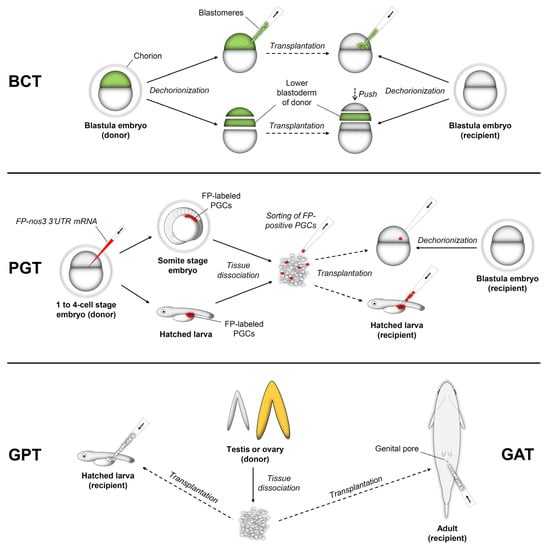### Detailed Caption for Infographic:

This infographic is divided into three distinct sections illustrating the processes and pathways involved in blastomer and embryo donor transplantation.

---

**Top Section: BCT (Blastomer and Embryo Donor Chlorinization)**

- **Step 1**: The section starts with "BCT, Blasto Embryo Donor Chlorinization" as a header.
- **Step 2**: It features two arrows indicating parallel processes:
  - **Dechlorinization to Blastomers Transplantation**: This pathway shows the dechlorinization process enabling the transplantation of blastomers.
  - **Lower Blastome of Donor Transplantation**: This pathway illustrates the transplantation of lower blastomes from a donor.
- **Step 3**: The section concludes with "Dechlorinization to Blasto Embryo Recipient," indicating a final step of preparing the embryo recipient through dechlorinization.
  
---

**Middle Section: PGT (Preimplantation Genetic Testing)**
  
- **Step 1**: The process begins with "PGT, FPNOS 3' UTR mRNA 1 to 4 Cell Stage Embryo Donor," focusing on early-stage embryos at the 1 to 4 cell stage.
- **Step 2**: The process can follow two pathways:
  - **Hatched Larvae**: The embryos transition to hatched larvae.
  - **Somite Stage Embryo**: Alternatively, the embryos reach the somite stage.
- **Step 3**: Both pathways lead to "Tissue Dissociation," where tissues are separated.
- **Step 4**: The dissociated tissues are then grouped together for "Sorting of FP Positive PGCs (Primordial Germ Cells)".
- **Step 5**: The sorted PGCs can follow two paths:
  - **Transplantation to Hatched Larvae Recipient**.
  - **Dechlorinization for Blasto Embryo Recipient**.
  
---

**Bottom Section: GPT (Gonadal Tissue Transplantation)**

- **Step 1**: This section starts with options for "Hatched Larva Recipient Transplantation" and "Adult Recipient Transplantation".
- **Step 2**: Both options converge on "Testes or Ovary Donor Tissue Dissociation".
  - The process involves dissociating the donor tissue from either testes or ovaries for further transplantation procedures.

---

The infographic meticulously outlines each step and pathway, from the initial stages of dechlorinization through various transplantation phases, providing a comprehensive understanding of these intricate biological processes.